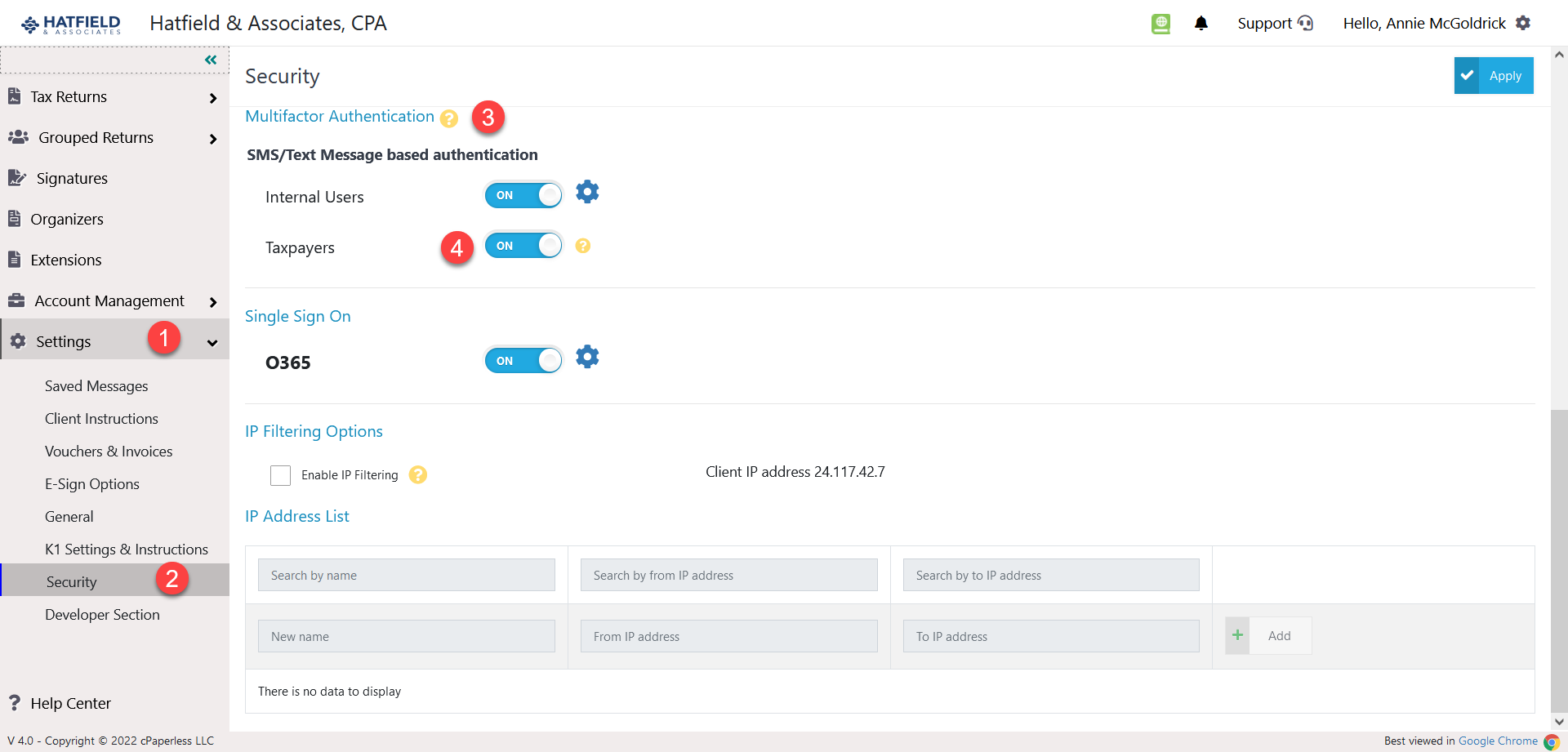The image displays a detailed interface from the Hatfield & Associates CPA website. At the top, a white bar features the blue Hatfield logo in the upper left corner, accompanied by black text reading "Hatfield & Associates CPA." On the upper right corner, there is a green button, a notifications bell, a support button with a headset icon, and a greeting message "Hello Ann Mcglockrick" followed by a settings icon.

Running down the left side of the image is a gray sidebar containing multiple tiles. These tiles are labeled: Tax Returns, Group Returns, Signatures, Organizers, Extensions, Account Management, Settings, Saved Messages, Chat, Chart Instructions, Vouchers and Invoices, E-Sign Options, General and KI Settings or Instructions, and Security and Developer section. Notably, the Security section has two notifications, while Settings has one.

In the center of the image, the Security section is prominently displayed, showing options with upward-pointing arrows. Additionally, the Taxpayers section contains four notifications, and the Multi-Factor Authentication section has three.